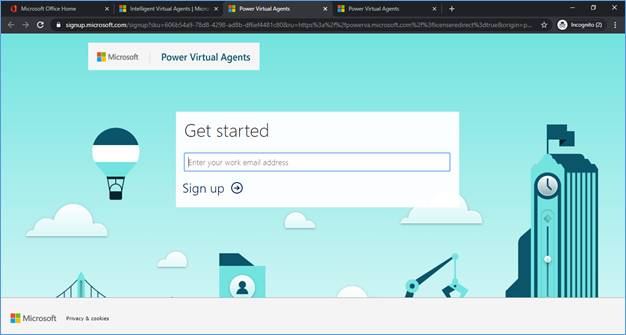This screenshot captures a browser window in incognito mode, displaying four open tabs titled: "Microsoft Office Home," "Virtual Agent," "Power Virtual Agent," and another "Power Virtual Agent" tab. The user appears to be initiating the setup process for Microsoft Office and Power Virtual Agent. The primary focus is on the "Get Started" page for Power Virtual Agent from Microsoft.

The webpage prominently features a "Get Started" button, followed by a field to enter a work email address and a "Sign Up" option, indicating this is the initial step for creating a Power Virtual Agent account. The site’s background showcases a dynamic blue graphic with various elements, including clouds, a hot air balloon, a clock tower, a crane, and the top of a suspension bridge, which add an engaging visual layer. The screenshot notably shows that the user is not logged into the browser, as evidenced by the incognito mode.